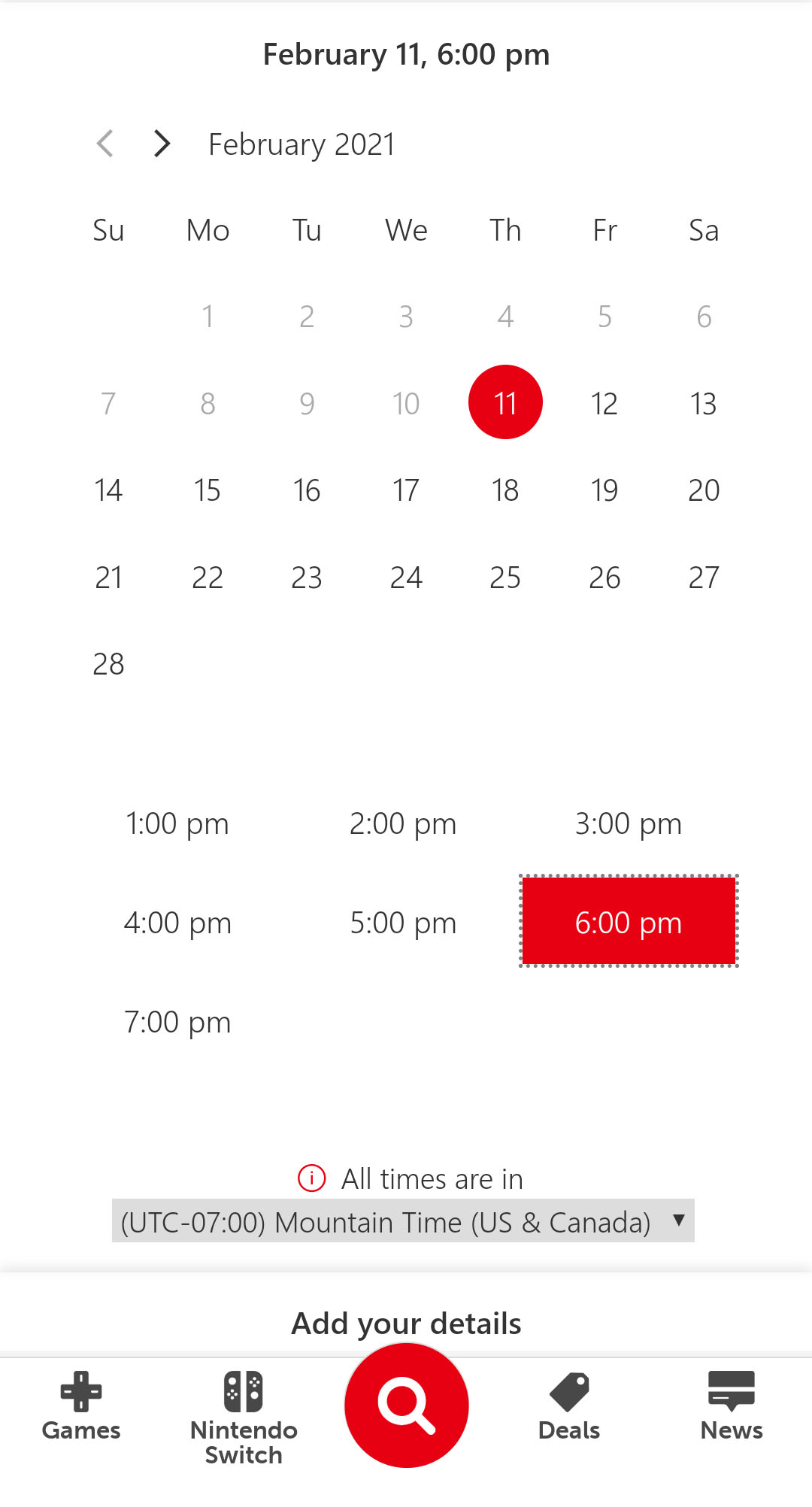At the top of the image, a grey line extends horizontally against a white background. Below this line, the text reads "February 11th, 6pm." Directly beneath this, there are symbols for "less than" (<) and "greater than" (>). The calendar displayed indicates it is for February 2021, laid out from Sunday to Saturday, with February 1st starting on a Monday and February 28th ending on a Sunday. Following the last day of the month, there is some blank space. Dates from the 3rd to the 11th are highlighted with a red oval. Below the calendar, the hours from 1pm to 7pm are listed sequentially. The 6pm time slot is emphasized with a red rectangular box around it. At the bottom, there is a red circle containing an exclamation mark, accompanied by text stating that all times are in UTC-0700 Mountain Time, US and Canada.